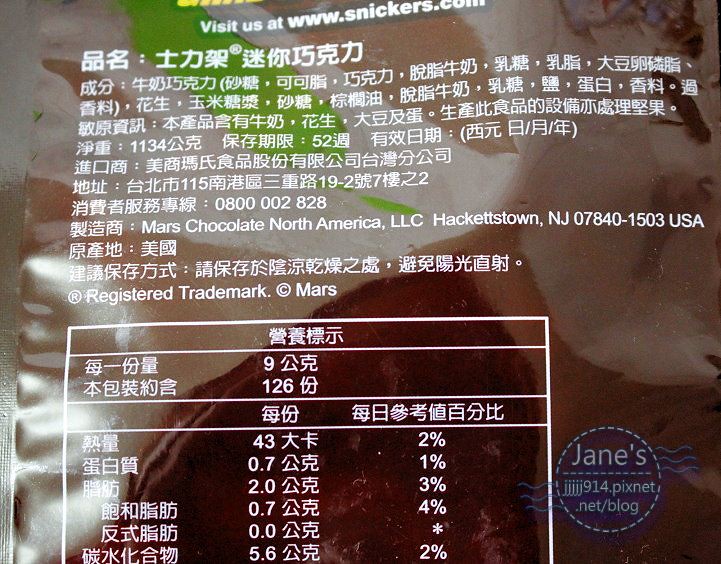This is an extreme close-up color photograph of the back of a Snickers package, specifically focusing on the nutritional facts. The package features both English and what appears to be traditional Chinese text. In English, it directs the reader to "visit us at www.snickers.com" and lists the manufacturer as Mars Chocolate North America, LLC, located in Hackettstown, New Jersey, 07840-1503, USA, noting it as a registered trademark of Mars. Numerical values such as "2%", "3%", "1%", and "4%" are present, indicating the nutritional percentages. Additionally, a watermark in the bottom right corner reads "Jane's", accompanied by "jjjjjj914.pixnet.net/blog" within a dotted circular outline.